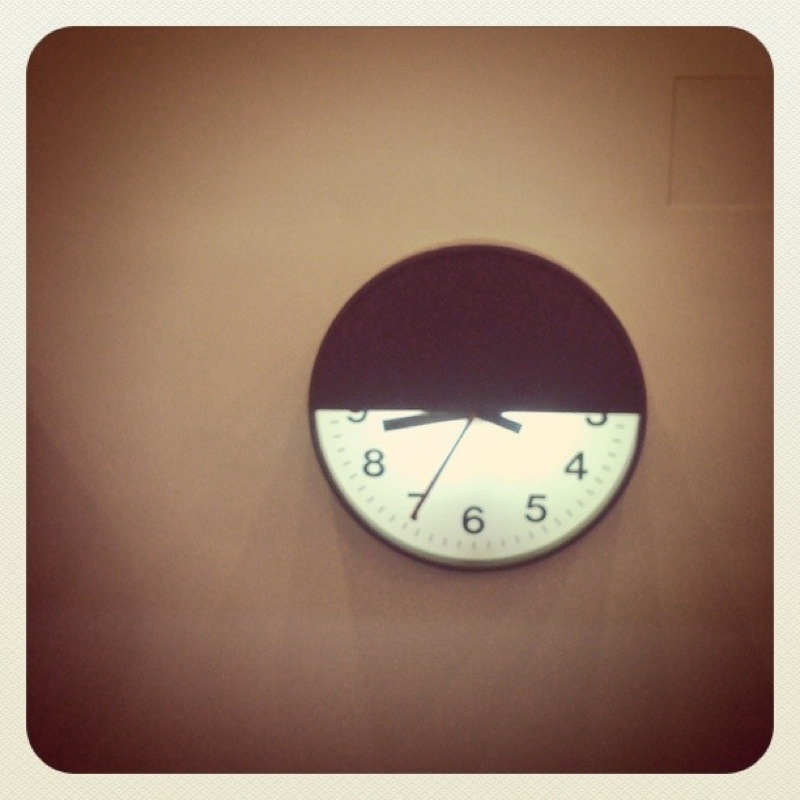The image showcases a vintage-style photograph with a tan border, featuring a light brown wall adorned with a round clock as the focal point. The upper half of the clock is obscured by a dark brown shading, which cuts through the numbers 9 and 3, while the lower half displays black numbers against a white background. All three clock hands—minute, hour, and second—are black, with the second hand resting on number 7. The upper right-hand corner of the photograph includes a built-in wall square. The overall color scheme of the image is in shades of brown, giving it a distinct, nostalgic feel.